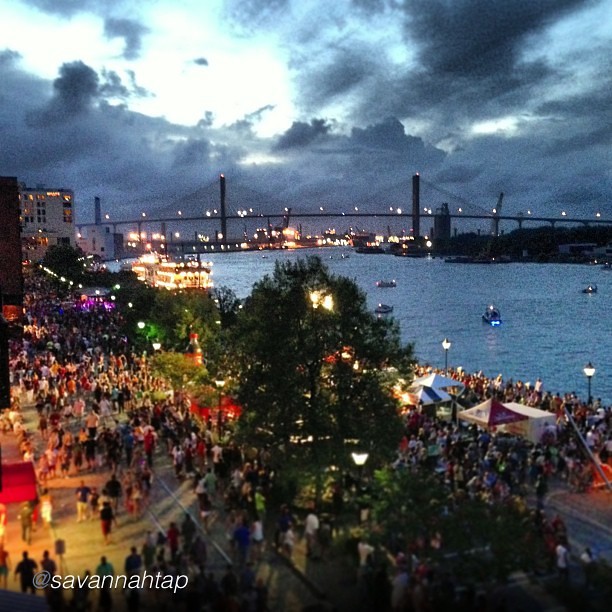This aerial photograph captures the bustling scene of a nighttime outdoor fair along the riverfront in Savannah. The lower-left corner features a watermark that reads "Savannah Tap," confirming the location. The fair is set on a city street adjacent to the riverbank, with the calm, blue water visible alongside. A large, illuminated bridge spans the background, its dark structure contrasting against the oncoming twilight sky, which is filled with dark blue, gray, and white clouds, suggesting either an impending storm or the transition to night.

The scene below is vibrant with activity. A large crowd mills around, seemingly unfazed by the looming clouds, enjoying the well-lit fair. Red tents line the street, creating a festive atmosphere. To the left, tall city buildings stand prominently, and the river itself is dotted with small boats, including a docked steamboat. Trees, some with lights draped over them, add a touch of greenery amidst the urban setting, and the crowd gathers in clusters, fully engaging in the festivities.